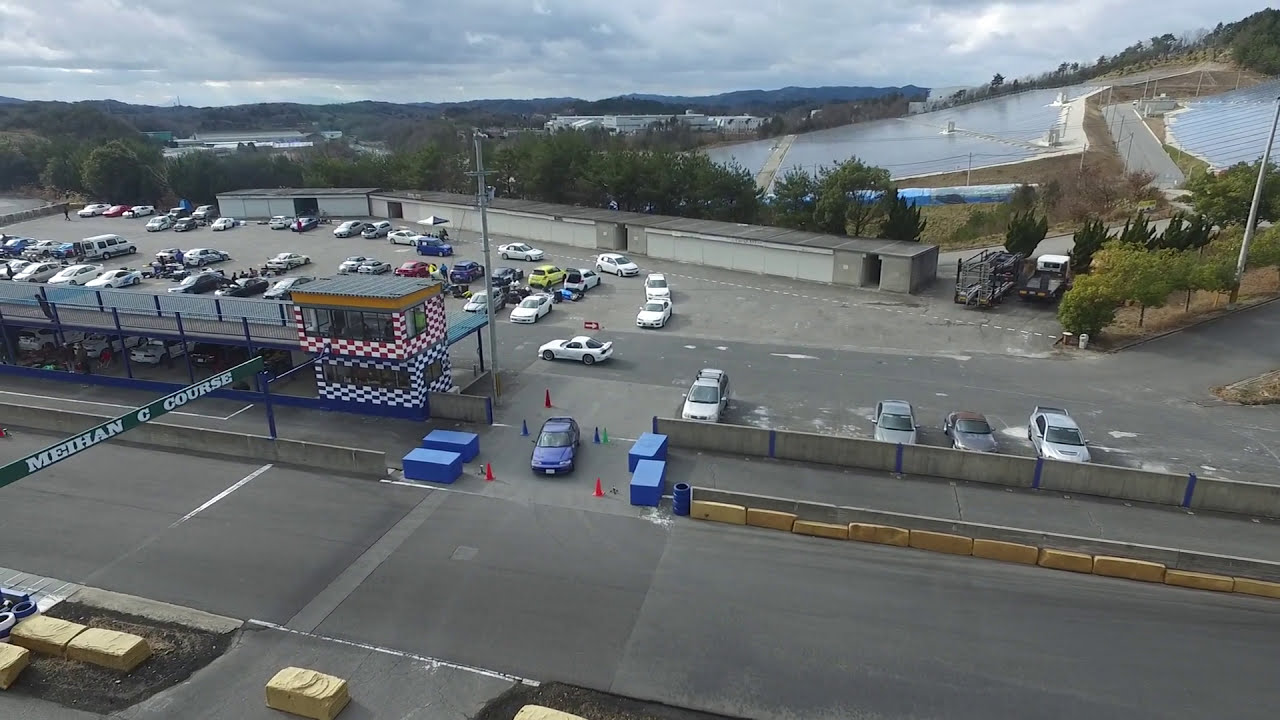The image presents a bird's eye view of an expansive outdoor area captured from a considerable distance. The sky in the background is cloudy and dim, hinting at an overcast day, though it remains daylight. Below the sky, there are stretches of trees and rolling mountain ranges.

Dominating the right-hand side of the image is an extensive water body, likely not the sea as there are no signs of a beach or coastal features. In the foreground, the scene is industrialized with a large, bustling parking lot filled with a diverse array of cars in various colors. Adjacent to this, a road cuts through the image horizontally.

Suspended above the road is a green sign with white block capitals reading "MEIHAN-C COURSE". This area appears to be part of a racetrack complex, evidenced by a black tarmac stretch running from the bottom right corner towards the left, accompanied by racing-specific podiums. The lower podium features blue and white checkered designs, while the upper podium displays red and white checks, both equipped with long windows.

At the bottom of the image, hay bales or beige bumpers line the raceway, designed to keep the cars on course. To the upper right, the landscape is covered with numerous flat solar panels glistening in the sunlight. On the left, the distant horizon reveals long rectangular buildings and clusters of trees. Behind these structures, there are rolling hills and additional buildings set against the cloudy sky.